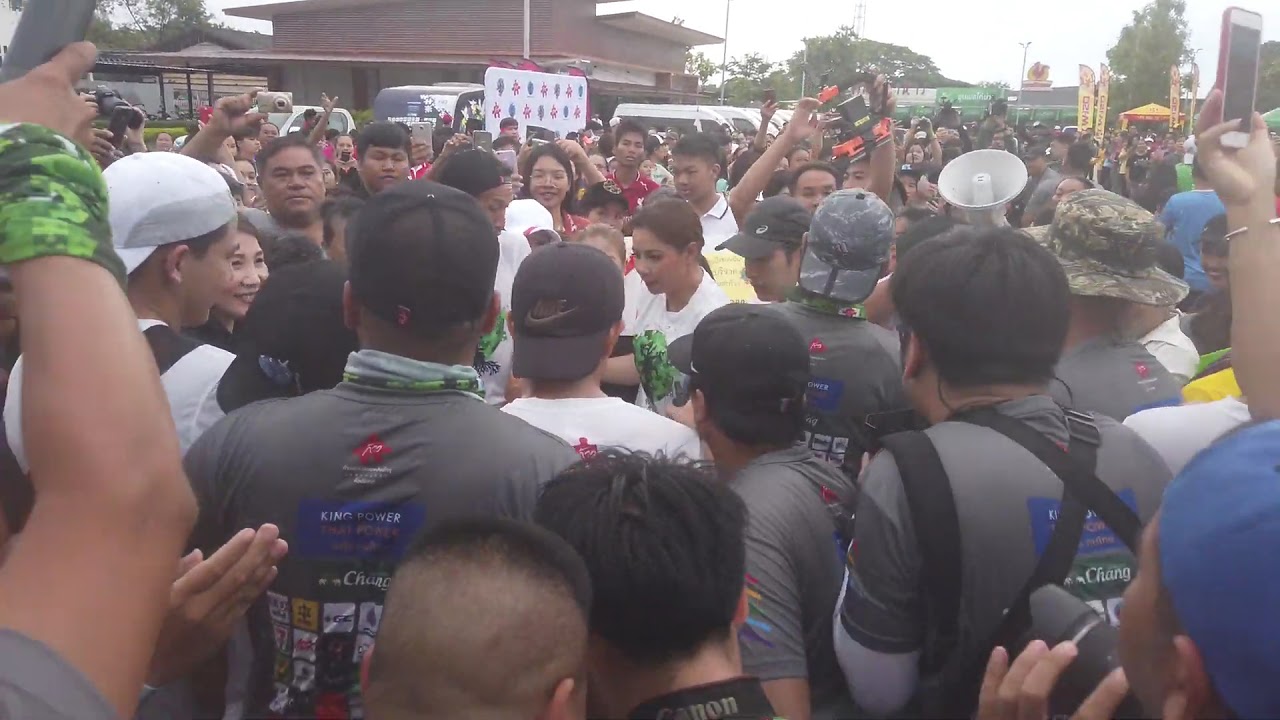This detailed color photograph, taken in landscape orientation from an elevated viewpoint, captures the bustling scene of a large crowd gathered outdoors in a town square or plaza. The setting is an Asian country, possibly Thailand or Singapore, as suggested by the architecture and script on a white sign in the distance. The image is vibrant with a palette of white, brown, green, gray, red, yellow, blue, and orange.

At the center of attention is a young woman with dark hair pulled back, dressed in a white t-shirt, holding a piece of paper or document. She is encircled by a diverse group of people: some smiling, others with their hands in the air, and a few holding signs and cameras, capturing the moment. Among the crowd, individuals sport casual attire—t-shirts, baseball caps, and backpacks. One person is notably holding a bullhorn.

In the background, a brown two-story wooden building and parked vehicles can be seen, with a few trees dotting the horizon above. The crowd, densely packed and animated, suggests the atmosphere of a celebrity event or public gathering, possibly even a protest. The image captures a lively moment of collective human activity in a public space, filled with energy and engagement.